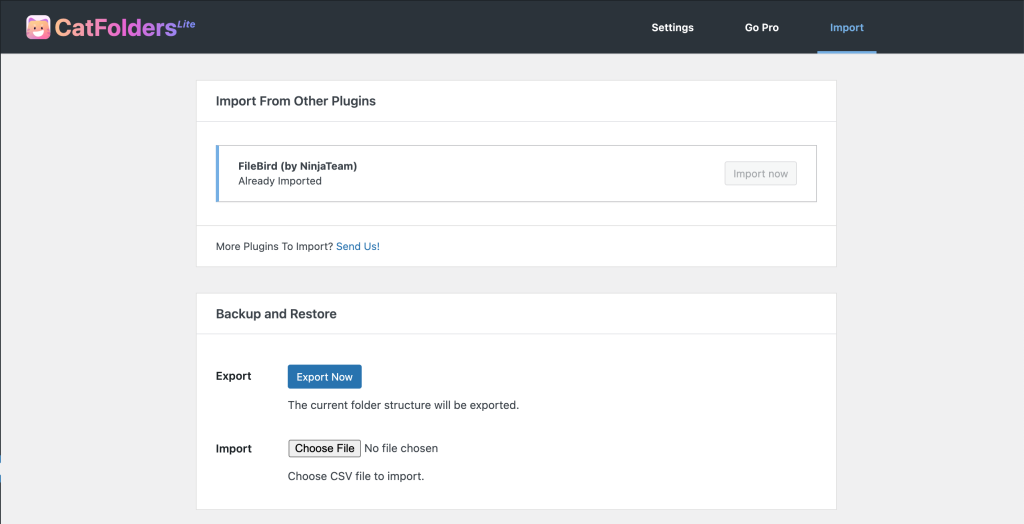The image appears to be a screenshot from a computer interface. At the very top, there is a black border. In the upper left corner, there's a small square icon featuring a smiling pink cat. To the right of this icon, the text "Cat Folders" is displayed, with "Cat" written in a pinkish color and "Folders" transitioning from pink to purplish-blue. Further to the right, there are three options labeled: "Settings," "GoPro," and "Import." The "Import" option is underlined and highlighted in blue.

The central part of the screen is dominated by a gray area with two white rectangles. The top rectangle reads "Import from Other Plugins" and includes a search bar labeled "File Bird (by Ninja Team)," followed by the status "Already Imported." Below this, there is an option that reads "More Plugins to Import" with "Send Us" highlighted in blue.

The second rectangle at the bottom is titled "Backup and Restore" and includes two main sections: "Export" and "Import." Under "Export," there is a blue button labeled "Export Now," accompanied by the text "The current folder structure will be exported." Under "Import," there is a "Choose File" button with the accompanying text "No file chosen" and an instruction to "Choose CSV file to import."